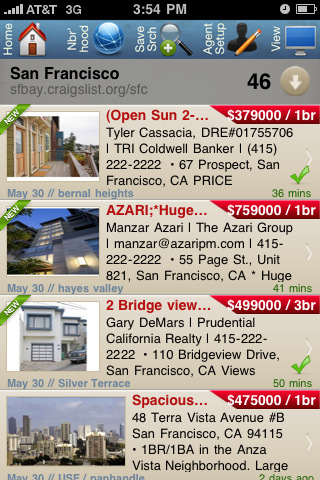A user is viewing an older property search website on their smartphone, specifically showing listings in San Francisco. The graphics on the site appear dated. The phone display indicates full reception with AT&T, 3G service, and the time is 3:54 PM. The battery is about 60% charged. The interface includes several icons: a house labeled "Home," a neighborhood light symbol next to a blue circle for "Safe Search," a magnifying glass for search, a person with a pencil for "Agent Setup," and a screen-view option.

The URL being accessed is "sfbay.craigslist.org/sfc46," with a dropdown arrow. Four property listings are visible:

1. The first listing features an image of a house and a "New" banner. It's priced at $379,000 for a one-bedroom located at 67 Prospect Avenue, San Francisco, with a timestamp and distance information of "36 May 30th, Bernal Heights." The layout appears unorganized.
  
2. The second listing is truncated, displaying "Azari, huge..." and requiring a click for more details. It’s a $759,000 one-bedroom property.

3. The third listing shows a $499,000 three-bedroom property.

4. The final listing, without a "New" banner, is priced at $475,000 for a one-bedroom and includes a photo of the city skyline instead of a house.

Overall, the listings are poorly organized, with the images and information not uniformly presented.